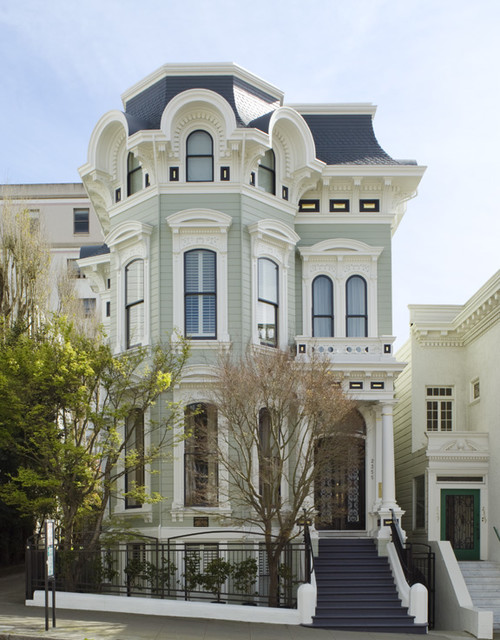This rectangular vertical photograph captures a beautifully refurbished old Victorian home, likely situated on a slanted street in a city like San Francisco. The majestic three-story house, including a basement floor with windows, features light gray vinyl siding and pristine white woodwork on the window and door trims. A rounded, turret-like section adorns one part of the facade, showcasing windows on all three sides, which adds an element of grandeur.

Ascending the dark-colored steps on the right side, one reaches the glass double front doors, framed in white with decorative panes. The ornate white columns supporting a small balcony above the entrance further accentuate its elegance. Surrounding the house, a white lower wall with black wrought iron fencing encloses a small front yard, hosting a couple of trees and some bushes. This area, alongside the sidewalk, integrates seamlessly with the similar-styled houses visible next door and behind, creating a harmonious neighborhood aesthetic.